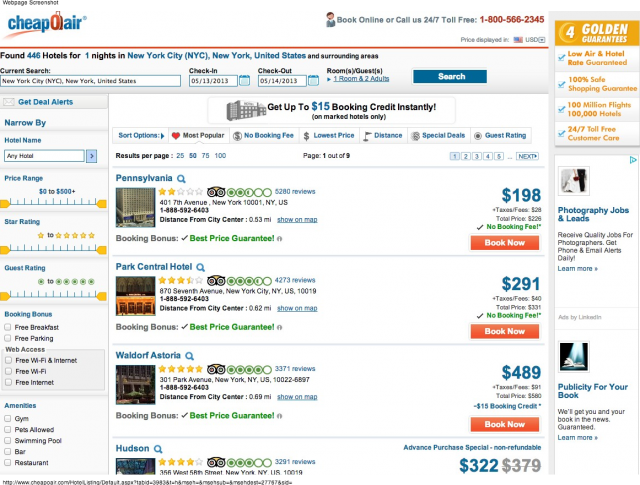Screenshot of a web page from Cheap O'Air, a hotel search website, featuring a busy and somewhat outdated design filled with information. The header section prominently displays the Cheap O'Air logo and includes an icon of a person alongside the text "Book online or call us 24/7 toll-free." Prices are shown in US dollars. In this specific screenshot, someone is searching for hotels in New York City for a one-night stay from May 13, 2013, to May 14, 2013. The search results reveal a total of 446 hotels, which are presented in a list format. Each hotel entry includes an image, review status, address, and price per night. On the left-hand side, there is a menu with multiple filtering options to refine the search results.